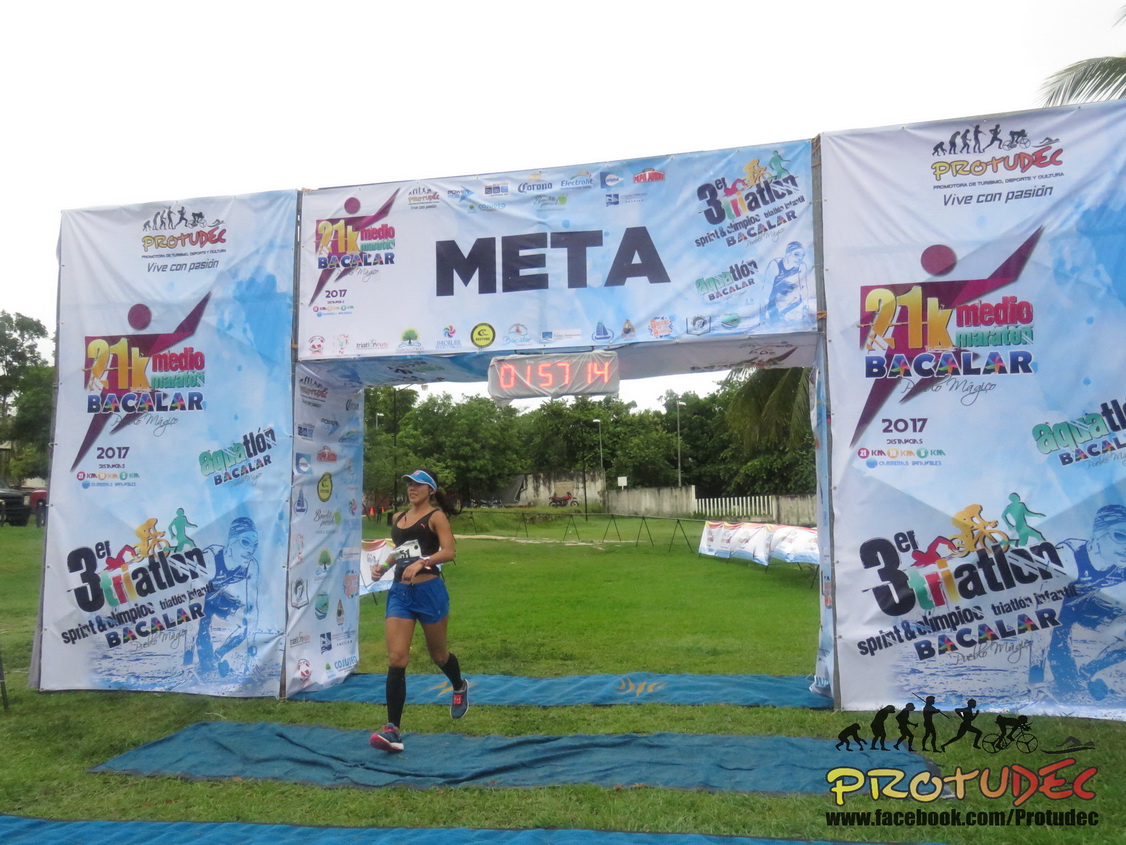The image captures a woman crossing the finish line of a strenuous race, likely a 21k marathon or triathlon, as indicated by the "META" and "21k" markings on the overhead banner. The event is highlighted by a digital clock displaying a completion time of 1 hour, 57 minutes, and 14 seconds. The race appears to be held in a non-American country, suggested by the multi-lingual sponsor logos adorning the portable finish line structure, which includes blue and white graphics of runners and various colorful sponsor emblems.

The athlete is sporting a blue visor, a black sports bra, blue running shorts, and gray running shoes. She also wears a white placard with an illegible number on her chest. The setting features a grassy field and a white fence in the background, and there seems to be no other runners visible, indicating she may either be leading or trailing in the race. A unique detail at the bottom right corner of the image includes a logo reading "ProTudeDEC" with a line art depicting the evolution of runners, accompanied by a URL for more information.